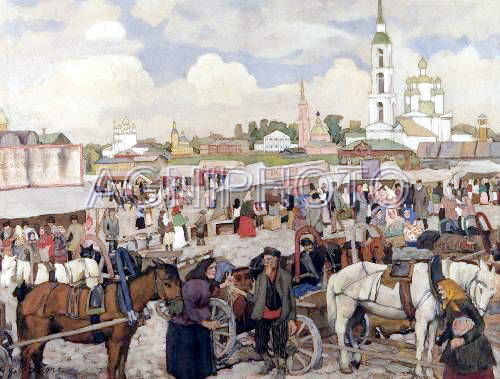This painting depicts a bustling outdoor market scene set in an old town or village, marked by an array of tents and stalls where numerous vendors and patrons are engaged in trading activities. In the foreground, two women, dressed conservatively in long skirts and long-sleeved tops with headscarves, lead a bay mule and a white mule, each pulling a cart. The marketplace is alive with groups of people milling about and interacting amidst the covered areas. The middle ground features additional market stalls and white tents, with people gathered and moving about. The skyline in the background showcases a diverse array of buildings, including a prominent tall, thin white structure with a spire and a large white building that could be a mosque or cathedral. The background gradually transitions into a residential area with a variety of colorful buildings of different shapes. Above this vibrant scene, the sky is dotted with poofy white clouds against a pale blue backdrop, adding to the picturesque and lively atmosphere of the market day. A watermark is situated directly in the center of the scene.